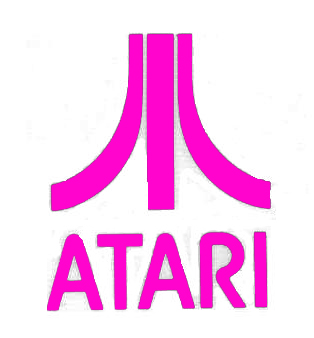The image displays the iconic Atari logo set against a white background. The design features a vertical pink line at the top center, flanked by two symmetrical, curved pink lines that resemble mirrored 'J' shapes on either side. These lines converge towards the central vertical line. Below the design, "ATARI" is written in hot pink, all-capital bubble letters. A subtle addition of gray shading appears between the lines, adding depth to the otherwise flat design.